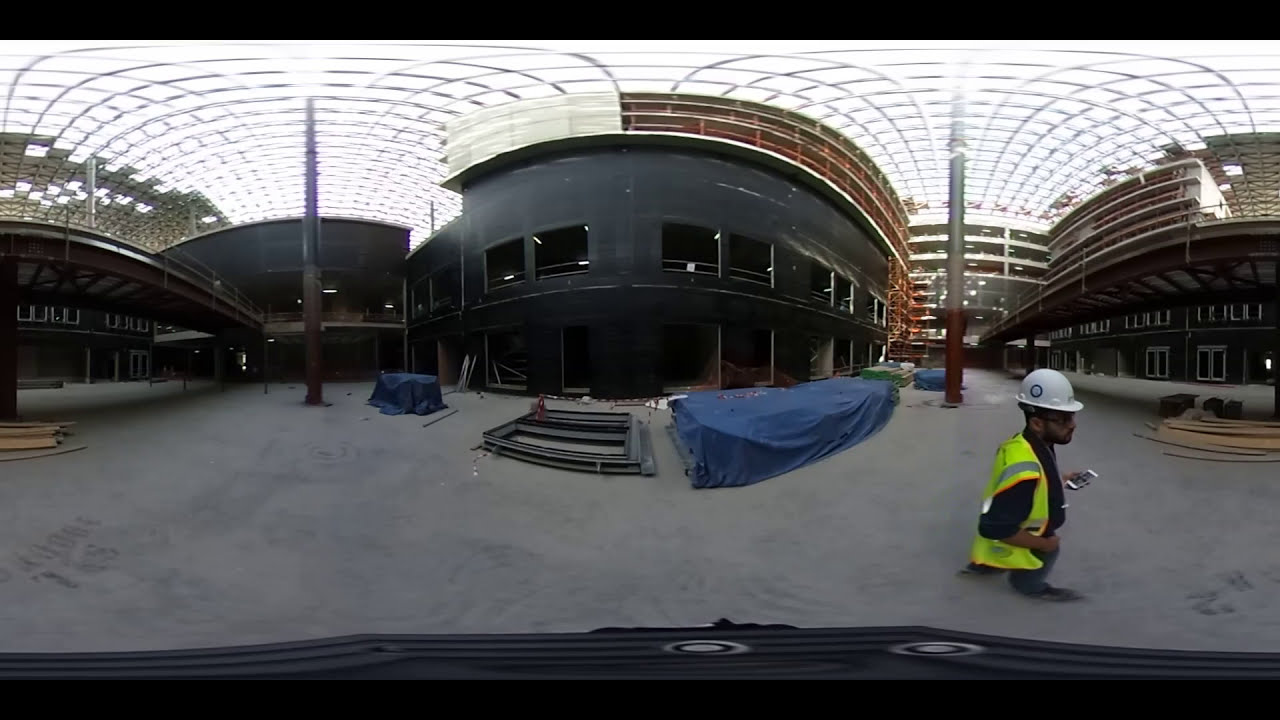The image depicts a panoramic 360-degree outdoor construction site featuring three buildings in a row. The middle building is distinctively black with numerous openings, likely indicative of an unfinished structure resembling a parking garage. On either side of this central building are two similarly structured buildings; the one on the right is grey with white framed windows and doors, matching the architectural style of the building on the left.

The structures are interconnected by a roof composed of metal wires, and the ceiling features arched skylights in square panels. In front of the central building, stacks of construction materials covered with blue tarps and pallets are visible. Between the buildings stands a pole with a red bottom and silver top.

In the foreground on the right, a dark-skinned construction worker with a beard is seen walking to the right. He is wearing a white helmet, a yellow safety vest, and appears to be holding a phone. The overall view is slightly distorted, likely due to the panoramic effect, and the scene is absent of any date or descriptive text.